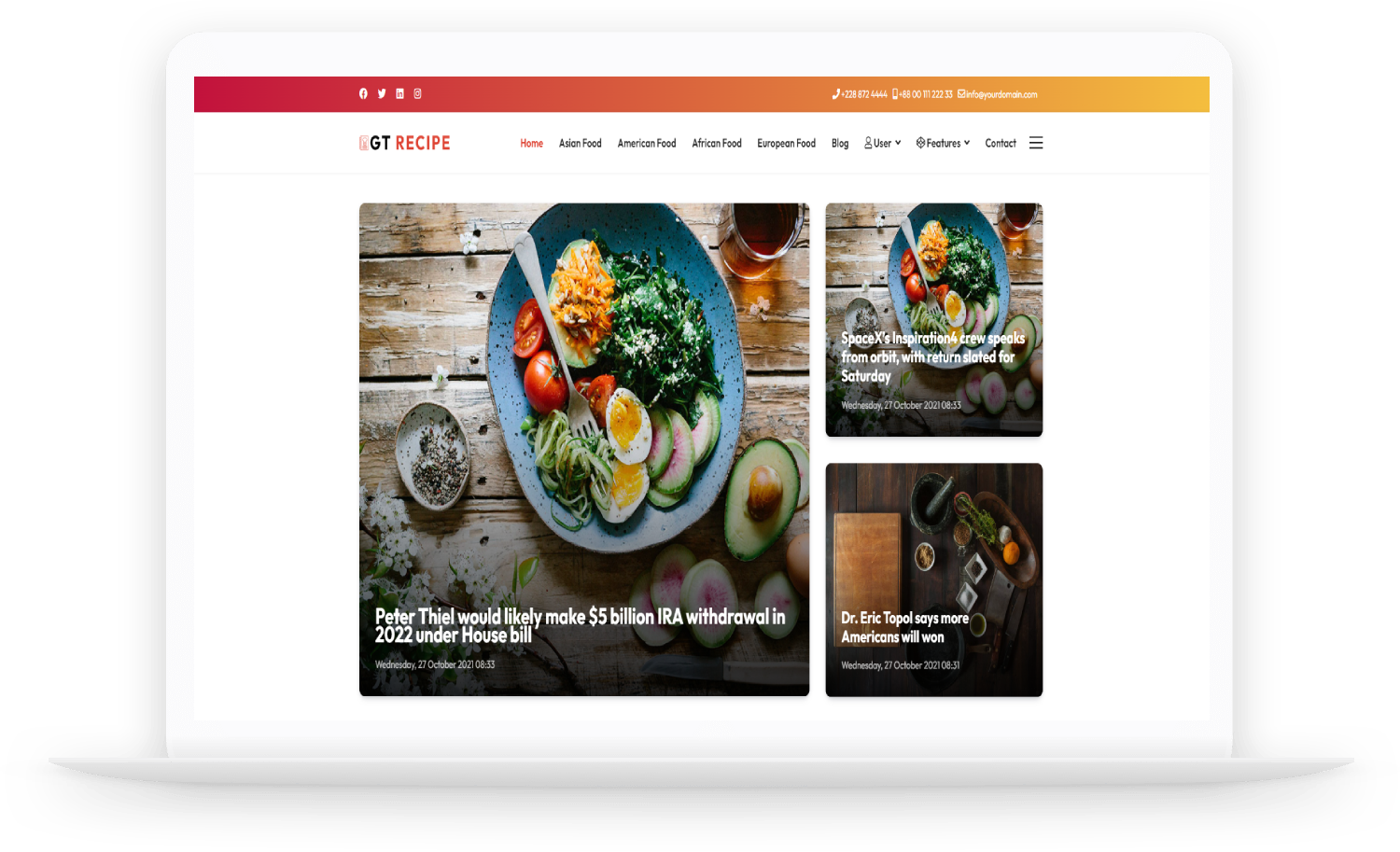The website image depicts the homepage of a culinary site named "GT Recipe." The design features a top banner that transitions from a red gradient to orange and includes various icons. The website title, "GT Recipe," is prominently displayed. Underneath, there's a navigation bar with the following categories: Home, Asian Food, American Food, African Food, European Food, Blog, User Section, Features [partly obscured], Contact, and a menu icon represented by three lines. 

In the main content area, there is a grid layout of three pictures. The left-side image is larger than the two on the right. The prominent left image is a top-down shot of a plate brimming with salad, accompanied by avocados and a drink, set on a table. The text overlay reads, "Peter Thiel would likely make five billion RIA withdrawal in 2022 under House bill." 

To its right is another section overlaid on the same food image. Below, there's an image of a table, captioned with "Dr. Eric Topo says more Americans will win." An additional but somewhat unclear image, which seems to be of books and perhaps food items, follows. The overall background of the website is white, ensuring that the content stands out clearly.